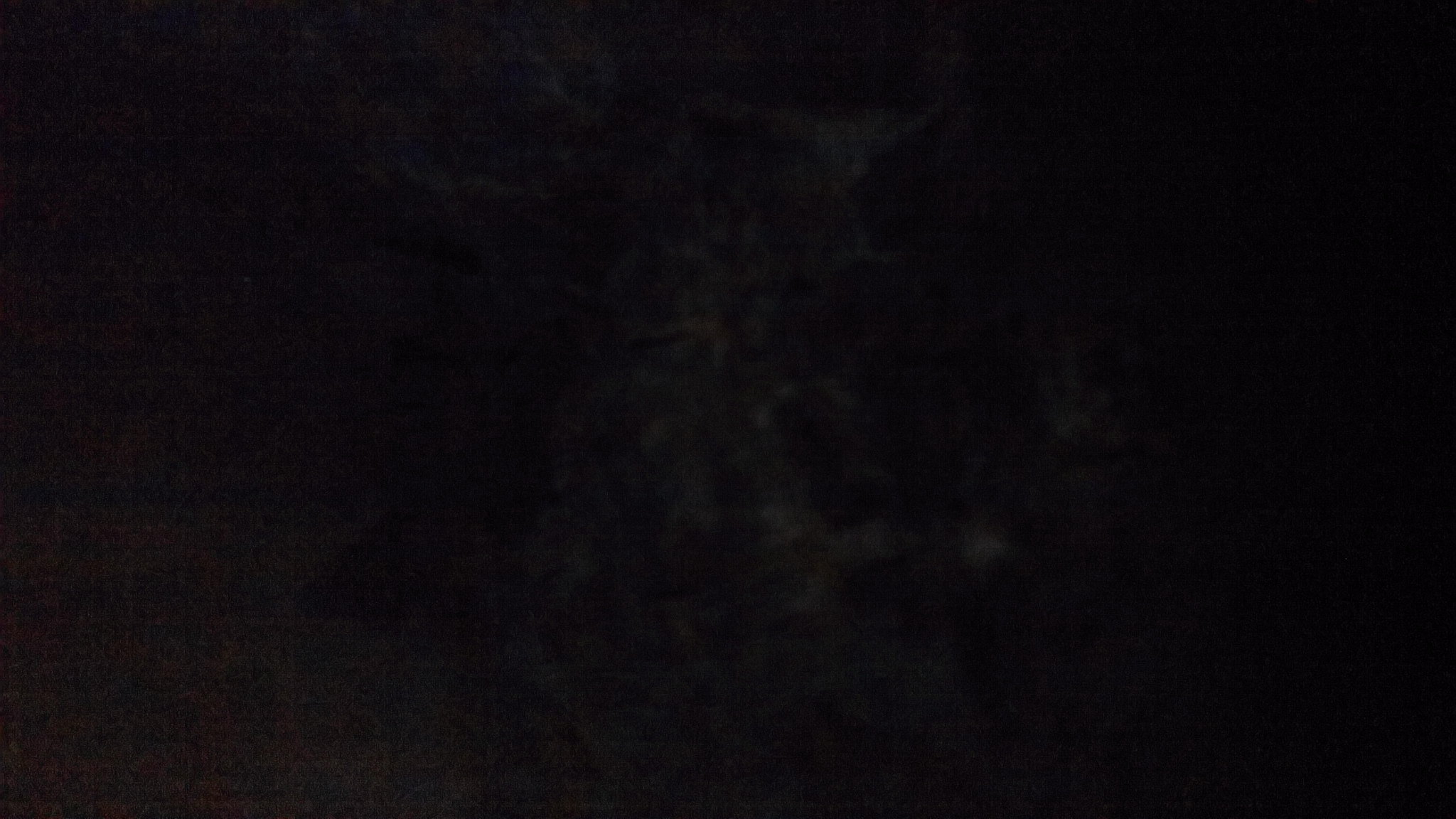This is a grainy, low-quality photo captured in landscape mode, dominated predominantly by a pitch-black background that makes up about 95% of the image. The photo's rectangular dimensions highlight a greater width compared to its length. Towards the left side of the image, the blackness slightly lightens, adding to the indistinct and obscure quality. Near the center, there is a very faint, wispy, greyish-white vapor or mist that lacks any discernible pattern or origin. The vaporous form seems almost hallucinatory, with some viewers speculating it might resemble the shadowy outline of an animal's face, such as a deer, wolf, or cat. However, the image remains largely indistinct and devoid of clear detail, rendering the central figure ambiguous and leaving much to the imagination.